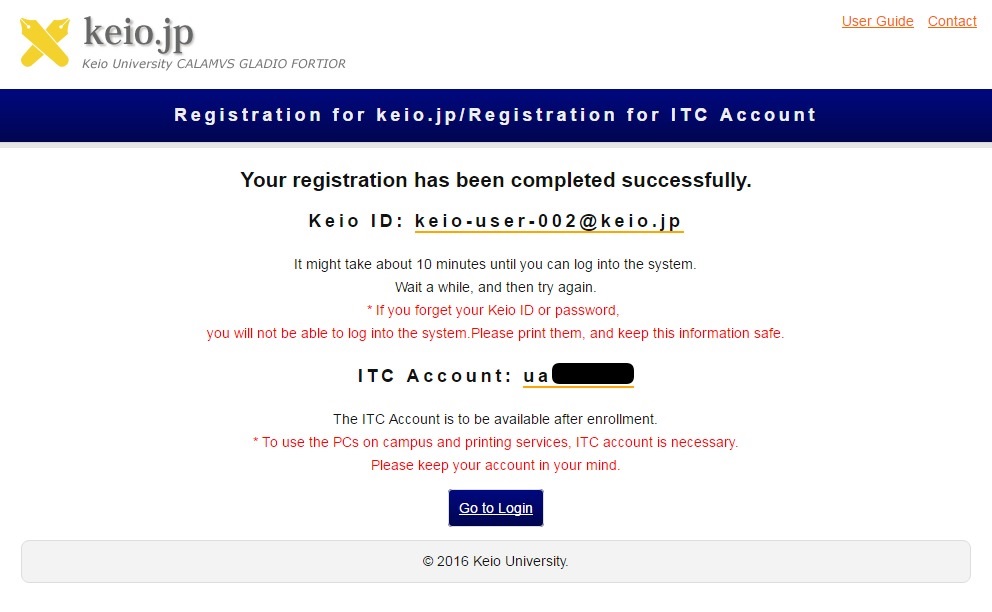The image displays a registration confirmation page from Keio University, specifically for creating an ITC account. The text is organized with various colors and highlights to emphasize important information.

At the top, the header reads "keo.jp, Keio University, Columbus, Gladio Fortier" in standard font. The main section of the page shows a message in blue text: "Registration for keo.jp/registration for ITC account." 

Below this, the text in black announces: "Your registration has been completed successfully." The user ID, formatted as keouser-002@keo.jp, is presented and underlined with a gold line for emphasis.

A subsequent message informs the user: "It might take about 10 minutes until you can log into the system. Wait a while and then try again."

An important warning in red reads: "If you forget your Keio ID or password, you will not be able to log into the system. Please print them and keep this information safe."

The ITC account details are partially redacted with "UA" followed by blacked-out text and similarly underlined with a gold line. 

Another notable message in red states: "To use the PCs on campus and printing services, ITC account is necessary. Please keep your account in your mind."

At the bottom of the page, there is a prominent blue button labeled "Go to login." Footer text indicates: "2016 Keio University."